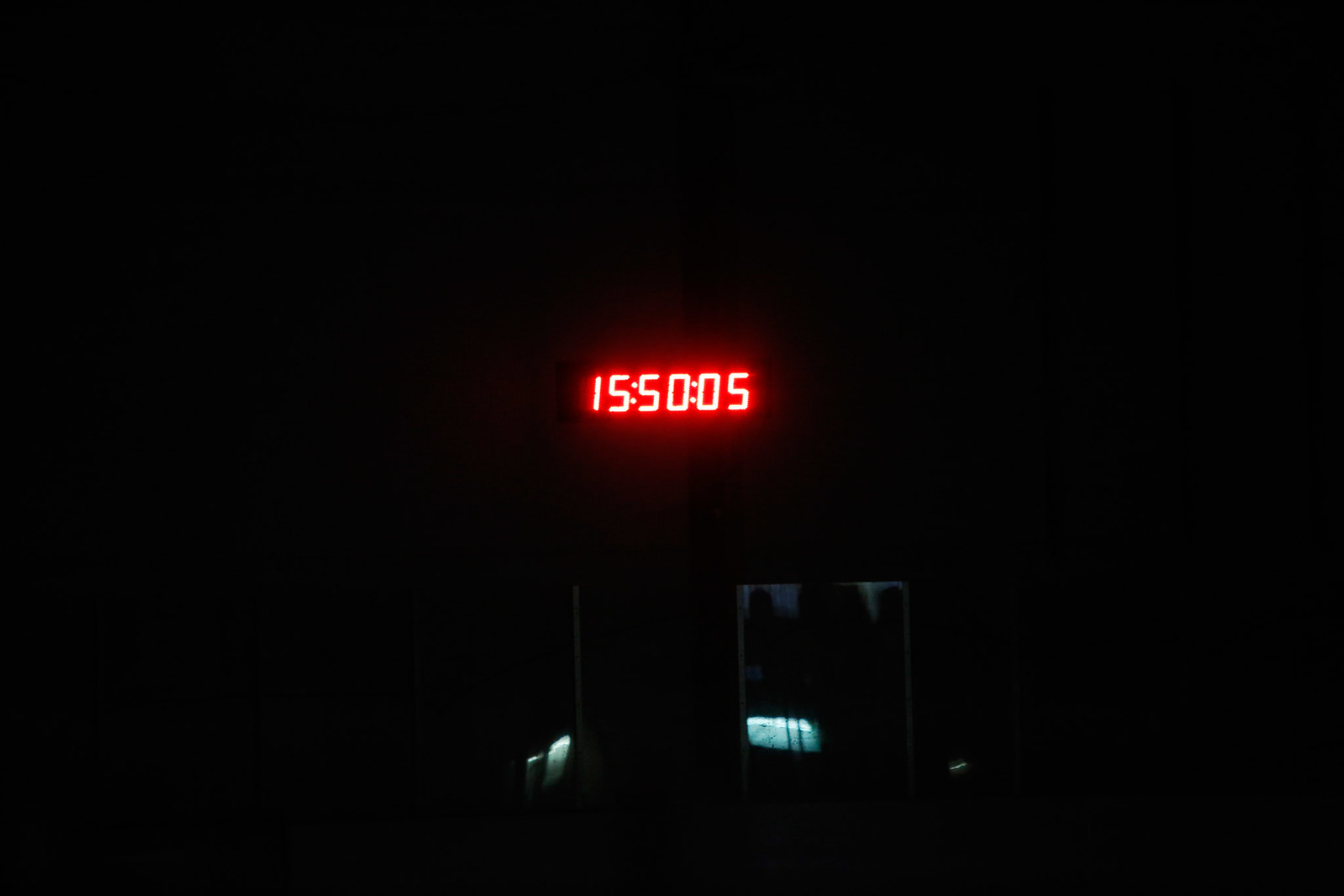The photograph captures a nearly pitch-black environment, with the primary focus being a bright red LED timer centered in the middle of the image. The timer displays "15:50:05," created by vertical and horizontal lines, suggesting a countdown from 15 hours, 50 minutes, and 5 seconds. This vibrant red glow starkly contrasts against the predominantly black background. Directly below the timer, there is a faint illumination that reveals indistinguishable details, possibly hinting at a greenish-blue object and the outlines of various items. On the bottom right, there appears to be a screen, while on the left, there seems to be a metallic piece resting on what looks like a desk; the object is black with silver trim. Despite these elements being barely discernible, they contribute additional depth to the otherwise dark setting.